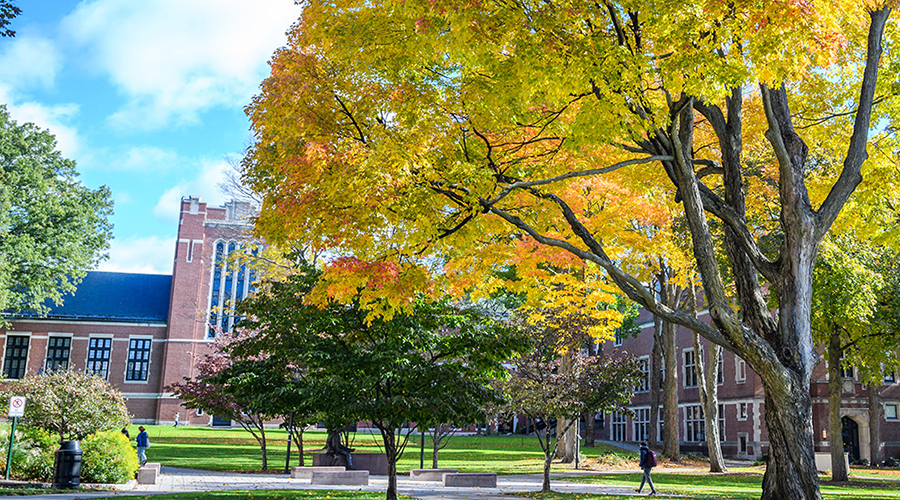In this vibrant photo of a university campus, the landscape is bathed in sunlight under a bright blue sky speckled with large, white clouds. The main focal point is a large, tall university building constructed from red bricks, featuring numerous large rectangular and arched windows. The building is topped with a distinctive blue roof that contrasts with the greenery below. In the foreground, a bright green, expansive grassy field is crisscrossed with stone pathways, one of which has several young people carrying backpacks, leisurely walking to their destinations. Scattered throughout the scene are a variety of trees in full autumn splendor, displaying a mix of yellow, orange, and a few light green leaves, with some trees on the right adorned with pink flowers. The right side of the image shows a closer view of a young man with a backpack, walking alongside a stone pathway. Stone benches placed strategically invite students to sit and enjoy the picturesque environment dotted by no parking signs. The overall scene encapsulates a serene and lively campus life amidst a beautiful fall day.